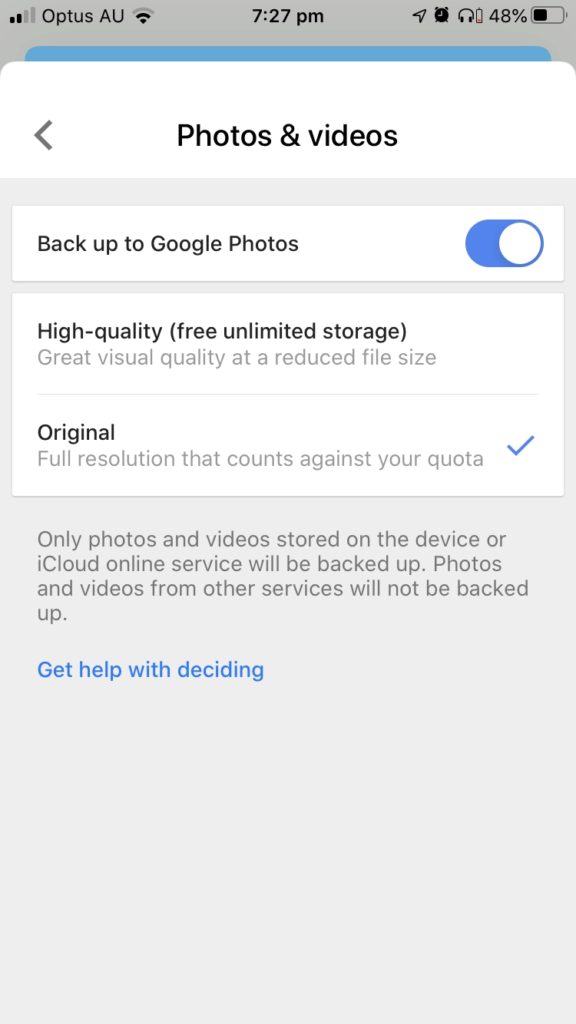The image displays a smartphone screen set to a configuration page for photo and video backup settings. The screen shows the following details:

1. **General Information:**
   - Date and Time: The time displayed is 7:27 PM.
   - Connection Status: The screen shows the status bars indicating cellular and Wi-Fi connections.
   - Battery Level: The battery is at 48%.
   - Device Label: 'Opus AU' at the top, indicating the device's name or perhaps a shorthand for the Australian region.

2. **Backup Options for Photos and Videos:**
   - The page title is "Photos and Videos" with a subheading, "Back up on Google Photos," which is toggled on.
   - **Backup Quality:**
     - High Quality: Offers free, unlimited storage with great visual quality at a reduced file size. This option is not checked.
     - Original Quality: Provides full-resolution backups but counts against the quota. This option is selected, marked with a blue checkmark.

3. **Instructions and Additional Information:**
   - A note explaining that only photos and videos stored on the device or iCloud (online service) will be backed up. Content from other services will not be included.
   - A blue hyperlink labeled "Get Help with this Setting" provides assistance.

4. **Design and Color Scheme:**
   - The background of the screen is primarily gray.
   - Text and interface elements are highlighted in white within horizontally elongated rectangles.
   - Colors on the screen include shades of gray, black, white, and two distinct blues: a teal blue and a more intense, real blue.

The overall design of this settings page is clean and functional, providing detailed backup preferences and pertinent information for the user.